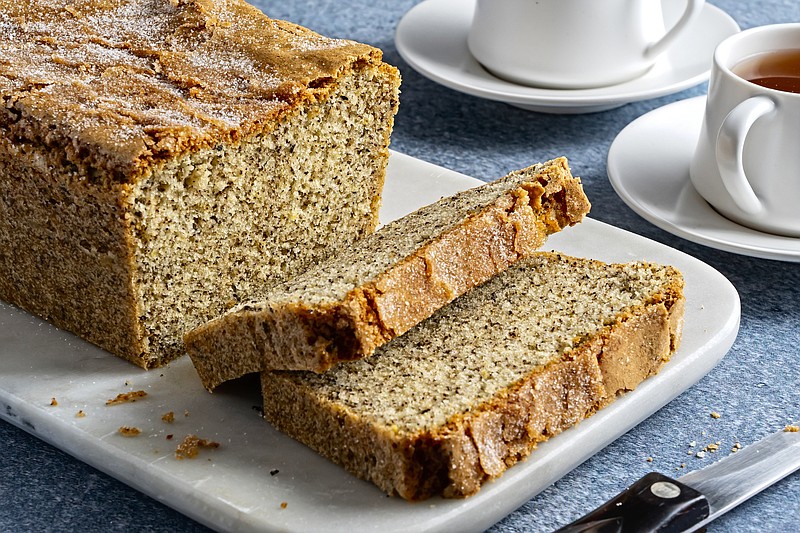An enticing horizontally-oriented image showcases a delectable loaf of banana bread, artfully seated on an elegant rounded rectangular white platter. The loaf has a warm brown crust with a subtle yellowish tone on the inside, indicative of its moist banana-infused texture. The top of the loaf is delicately dusted with powdered sugar, lending an appetizing touch. Two slices of the bread, about an inch thick, have been cut and are arranged neatly beside the remaining loaf. The surrounding scene includes a black-handled cutting knife resting on the table below the platter, its blade adorned with a few crumbs, as well as additional crumbs scattered on the platter and table. Behind the platter, partially visible, are two white cups on matching saucers, each filled with a dark beverage—likely coffee or tea, with one cup's contents visible. The setting suggests a tranquil moment of enjoying a comforting snack and coffee on a bluish-gray table, accented by the warm, inviting presentation of the banana bread.